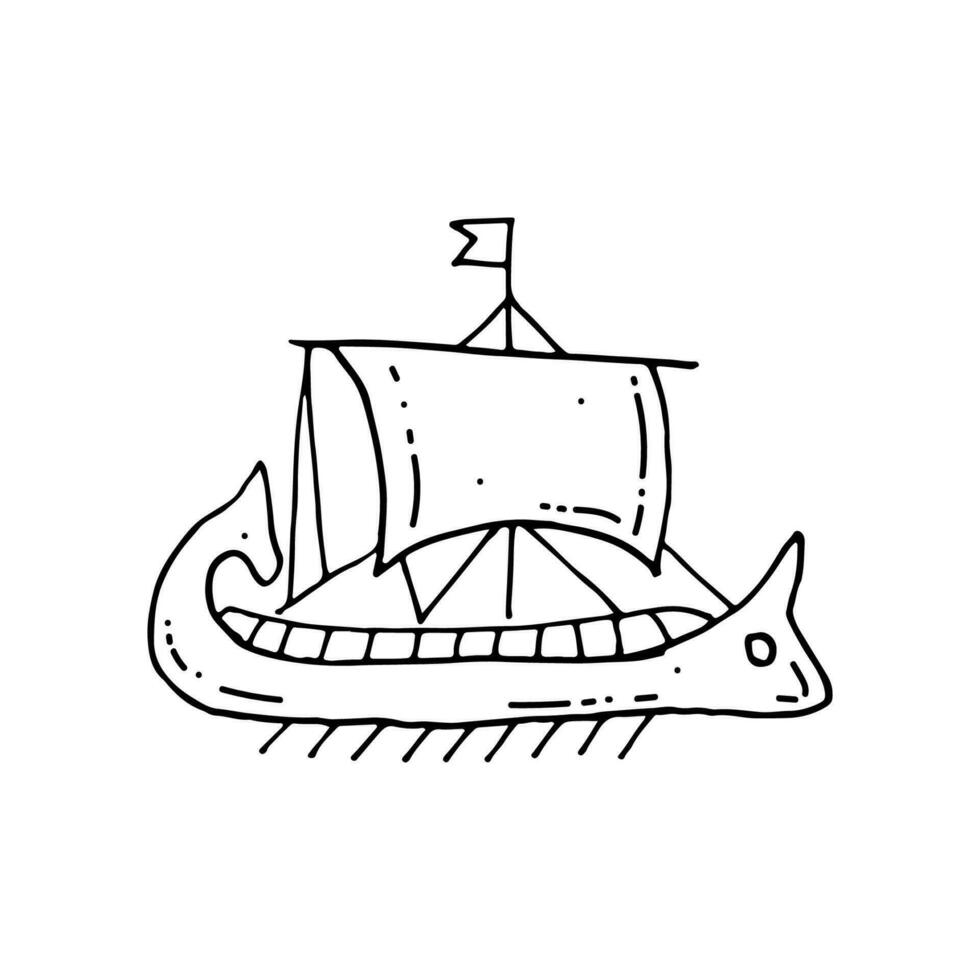This black-and-white line drawing depicts a minimalistic, ancient sailing ship, possibly Viking in design, as suggested by several distinct characteristics. The ship, viewed from the side, features upward-curving ends that bear simple, dragon-like faces. It is equipped with a series of oars protruding below the deck for propulsion, alongside a single, large rectangular sail that appears to be catching the wind, giving the vessel a sense of motion from left to right. Atop the sail, a notched flag flutters, adding to the dynamic feel of the scene. The ship's design, including its dragon-head prow and stern, indicative seating rows, and intricate details like the building-like structure amidships, evoke a sense of historical craftsmanship. Notably absent are any human figures or water, focusing attention entirely on the ship itself.